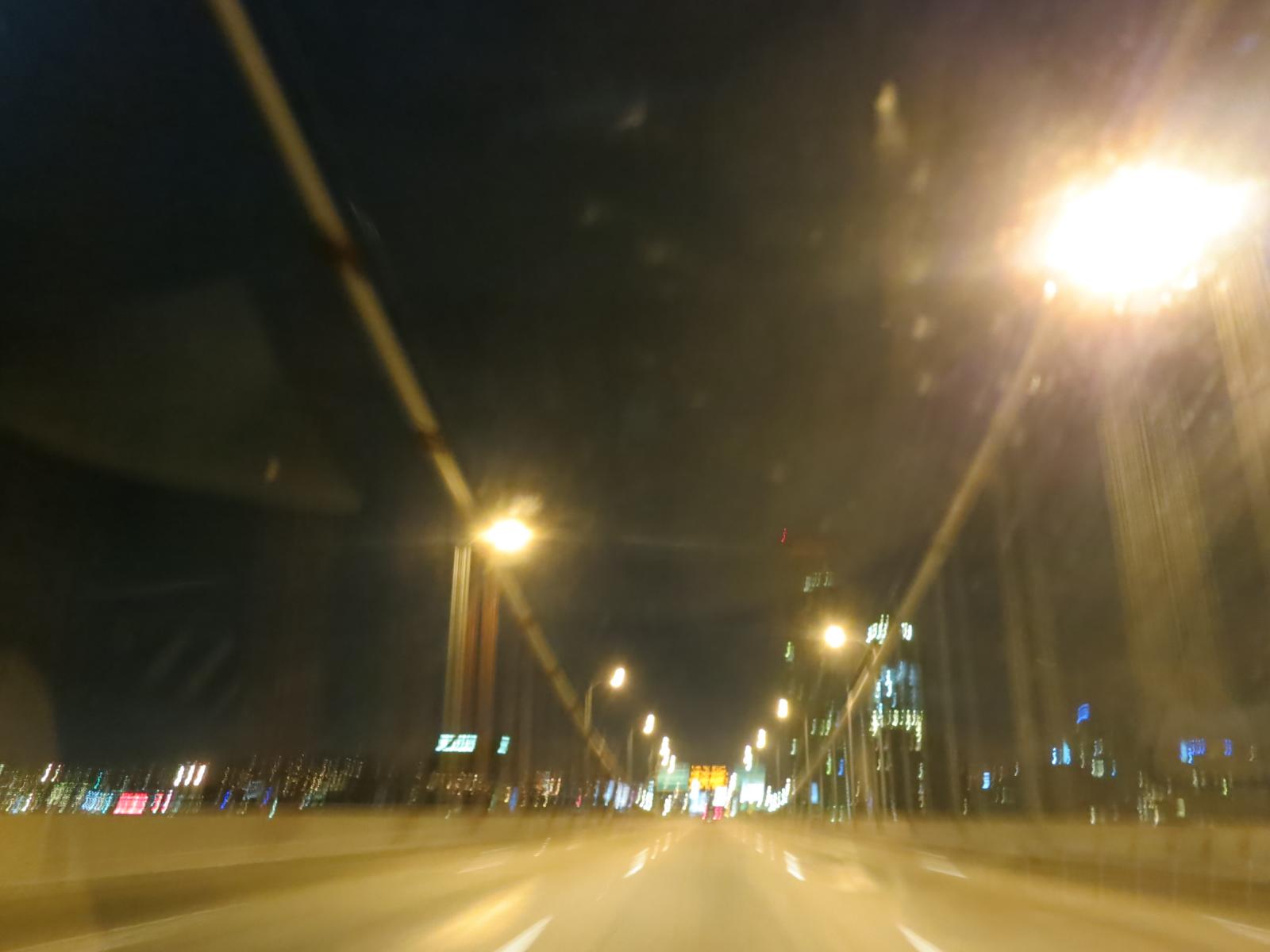This image features a striking, illuminated bridge extending towards a vibrant cityscape, reminiscent of Manhattan. The skyline in the distance is adorned with tall, glimmering buildings, though they appear slightly blurred, perhaps conveying the lively energy of the city. The bridge, also softly blurred, is adorned with a series of lights that cast a gentle glow on its structure and the three-lane roadway below. The absence of vehicles on the bridge suggests the photograph was captured in the middle of the evening, during a lull in traffic. Prominently displayed is a sign at the entrance of the bridge, possibly indicating construction information or toll costs. The image likely was taken from within a vehicle, evidenced by the perspective, and altered by the photographer to enhance the blurriness, adding an artistic touch to the scene.